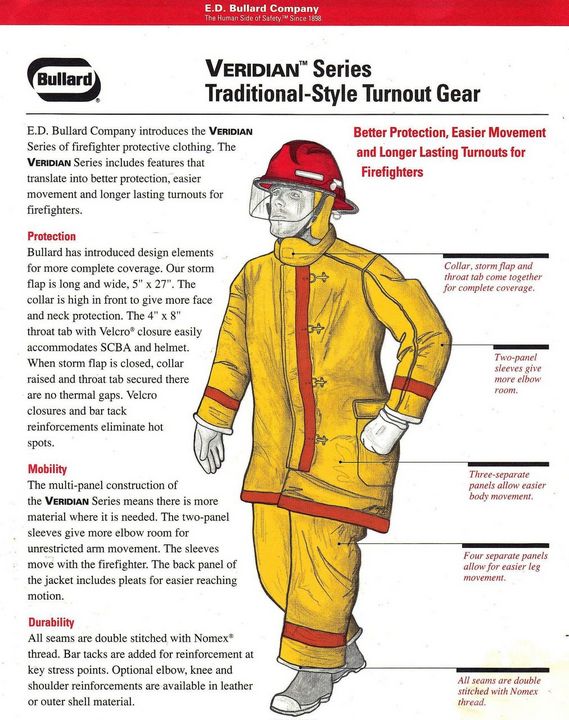The image is a detailed advertisement for a firefighter's suit from the Bullard Company's Viridian Series Traditional Style Turnout Gear. The ad is laid out on a largely white background with black text and a red header at the top. This red header reads "E.D. Bullard Company." Directly below, a white border bears the Bullard logo alongside the product name, "Viridian Series Traditional Style Turnout Gear," centered in black text. The image prominently features a firefighter, situated in the center, dressed in a yellow coat and pants with red stripes and a red helmet. The firefighter appears to be in mid-stride, walking towards the 7 o'clock position. Surrounding the firefighter, text blurbs point to different parts of the gear, detailing its features. Key descriptors include recommendations for better protection, easier movement, and longer-lasting turnout gear for firefighters. On the left side of the page, several paragraphs are categorized under headers such as "Protection," "Mobility," and "Durability." These sections expound on the suit's features, mentioning double-stitched seams with Nomex thread and reinforcements at critical stress points.